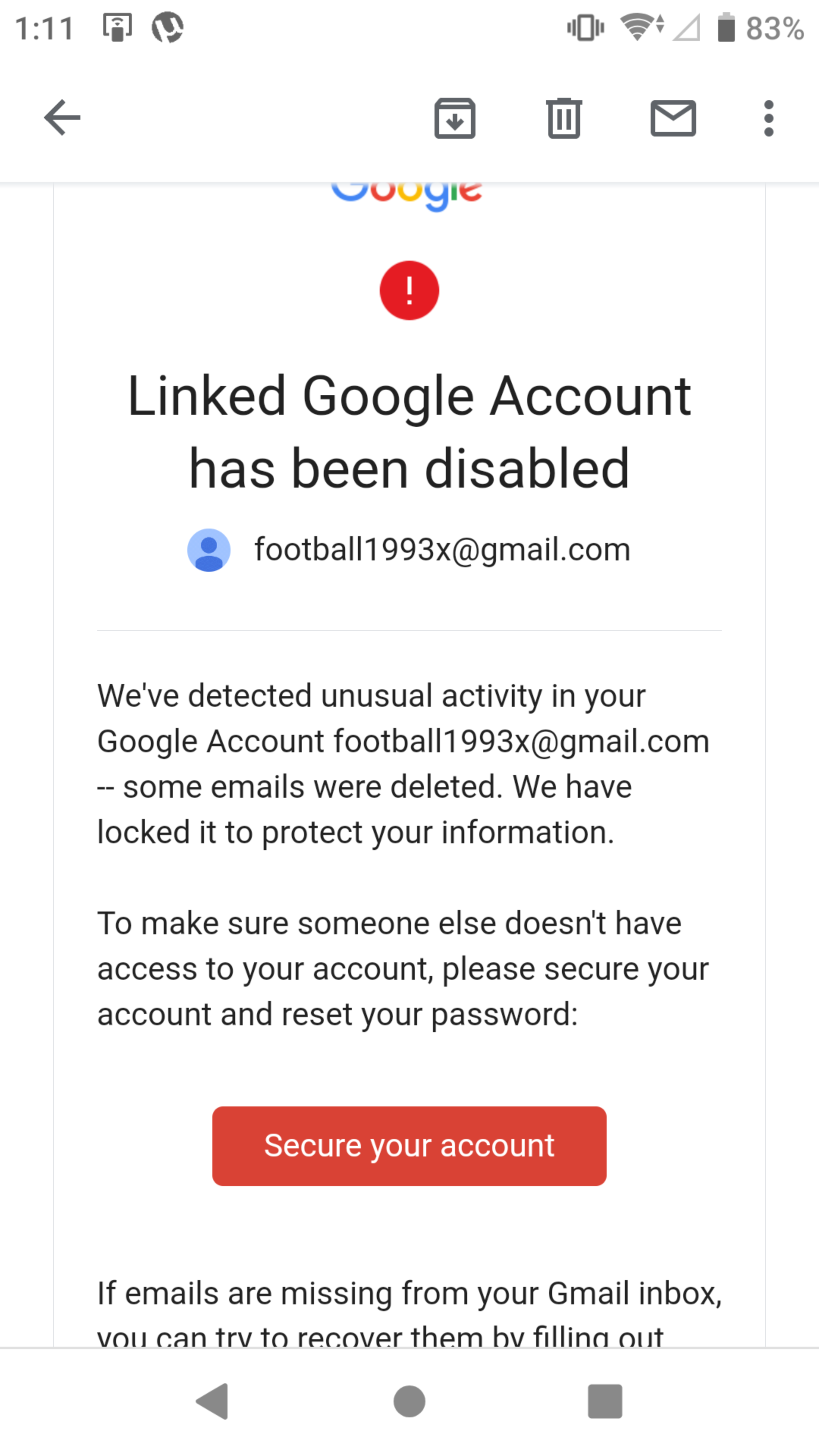The image shows a smartphone screen displaying a Kukli Mail page. At the top center, the logo "Kukli" is presented with letters in various colors: the first 'K' is blue, 'u' is red, the second 'K' is yellow, 'l' is blue, 'i' is green, and the surrounding design elements are red. Below the logo, there's a red circular icon with a white exclamation mark in the center, indicating an alert.

Further down, the email text, written in black, states that the linked Kukli account with the username "football1993x@gmail.com" has been disabled due to detected unusual activity. The email informs the user that some emails were deleted and the account has been locked to protect their information. It advises the user to secure their account and reset their password to prevent unauthorized access. Below this message, there's a prominent red button with white text that reads "Secure Your Account," intended for account recovery.

At the very bottom, the email mentions that if emails are missing from the user's Gmail inbox, they can attempt to recover them, though the message cuts off there. The email background is white, and the top of the screen features grey icons for archive, delete, inbox, and menu options. Overall, the design is clean and focuses on alerting the user to take immediate action to secure their account.